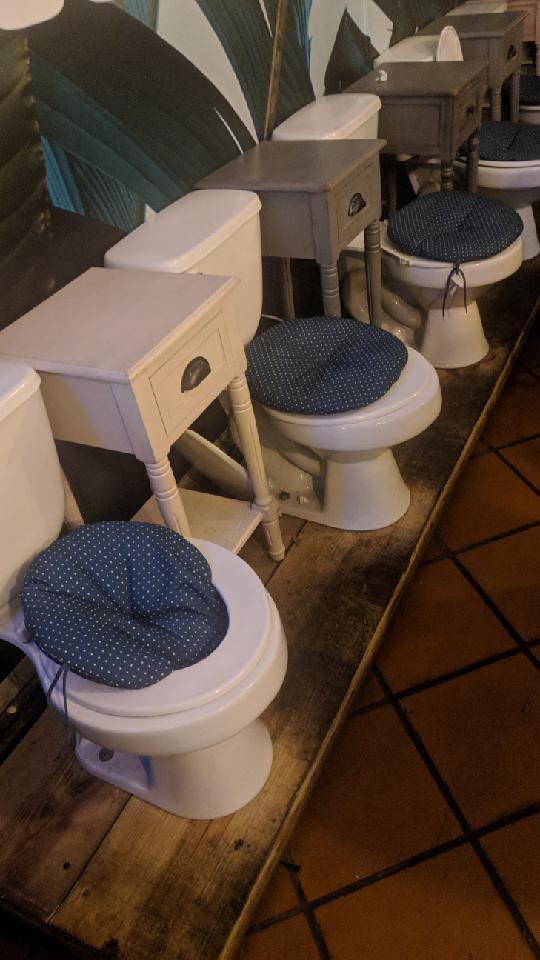The photograph showcases an unusual restroom interior with a row of white toilets meticulously lined up on a long wooden platform. Each toilet features a round blue cushion on the closed seat. There's a small, one-drawer table, resembling a nightstand, positioned between each toilet—three of them in light gray and one in white. The platform rests on a wooden floor, and just ahead lies a reddish-brown terracotta tile floor with prominent black grout lines. The back wall is adorned with an eye-catching mural featuring large, dark green and white plant-like designs, lending a tropical ambiance to the scene. This intriguing setup appears to be a display, possibly within a showroom.